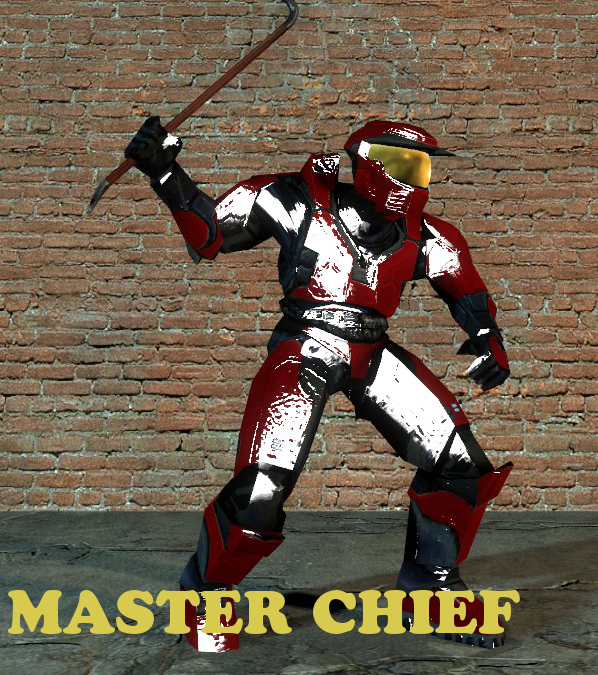In the image, the person is dressed as Master Chief from the Halo video game series, but with a unique twist. The costume consists of a shiny, red and black suit of armor that covers the entire body from legs to feet, complemented by a matching red helmet featuring a yellow visor. The character dons black gloves and is holding a brown crowbar with black tips in the right hand, poised as if ready to swing it. The scene is set on a grey, stone-like floor, with a backdrop of brown brick walls. At the bottom left corner of the image, the text "Master Chief" is prominently displayed in yellow letters. This fan-made art appears to blend elements from the Halo series with the Half-Life video game, offering a creative and detailed crossover depiction.